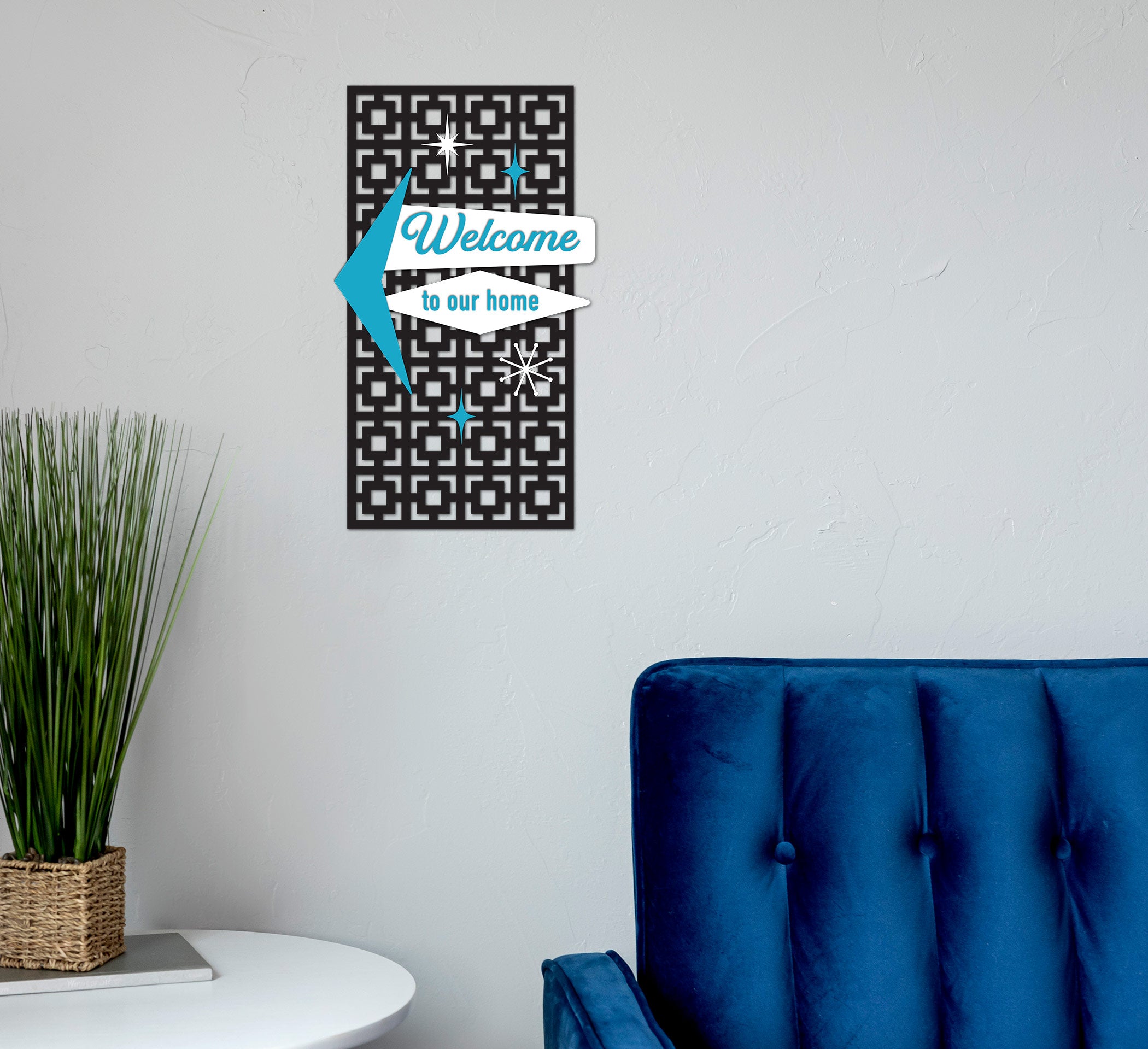The photograph captures a stylish, cozy corner of a living room enhanced by bright and distinctive elements. Dominating the right side of the image is a luxurious cobalt blue velvet couch, its plush back cushion partly visible and exuding a slight sheen. Adjacent to the couch is a compact, white, circular end table. On this table sits a vibrant green plant in a brown wicker basket, looking lush and healthy with straight green prongs. The backdrop features a white plaster wall with a textured surface, adorned with a black, square-patterned poster resembling the iconic "Welcome to Las Vegas" sign. The sign prominently features four stars—two white and two blue—and displays the text "Welcome to Our Home" in a light blue font on a white background, with an arrow pointing to the left of the text. This corner presents a balanced blend of comfort and personality, making it a welcoming part of the home.